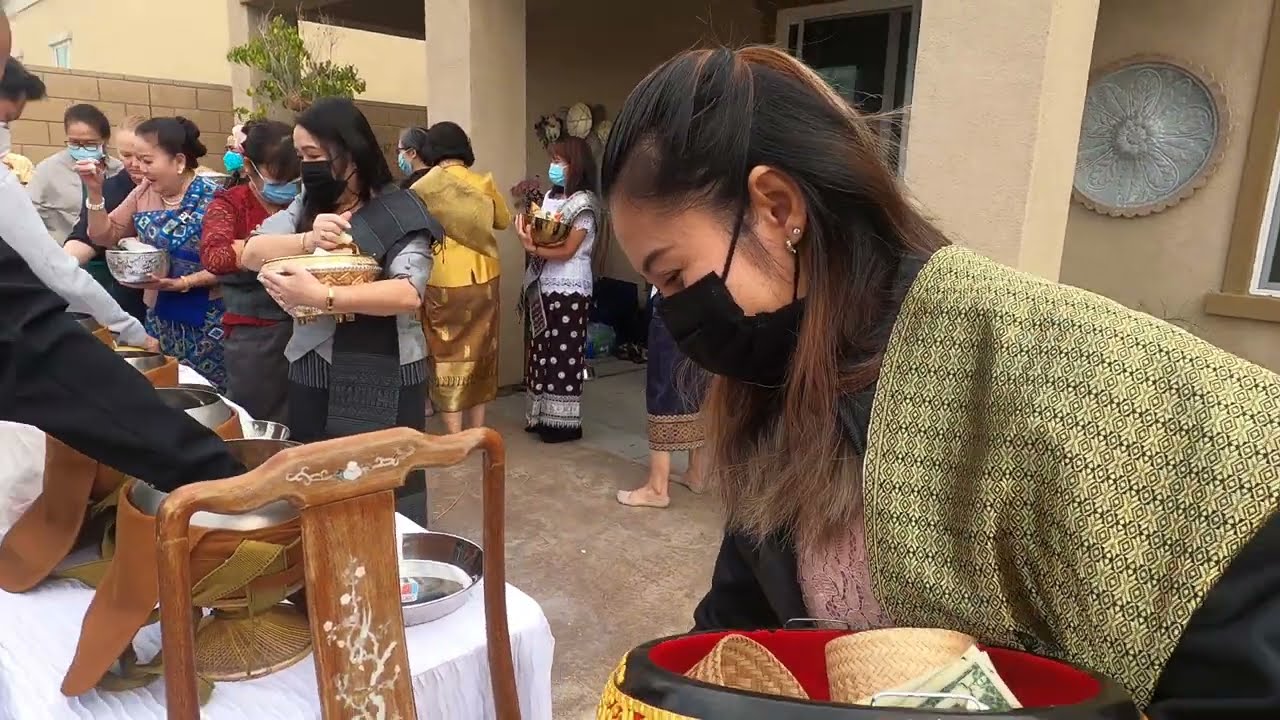The image captures a busy outdoor market, possibly located in an Asian country. Prominently in the foreground to the right, a light-skinned woman with dark brown hair, partially masked in black, is seen wearing a greenish scarf with black patterns over a black dress. She holds a large decorative basket containing dollar bills and smaller woven bowls. This woman features small hoop earrings and a tiny diamond earring above them. To her left extends a white table covered with a tablecloth, adorned with several large bowls. The table appears to be part of a food distribution setup where people's arms reach across to serve or receive items.

The background reveals twelve individuals, most of whom are women wearing long, multicolored dresses or robes, and either blue or black masks. Half of the women are holding decorative bowls, and a few are pointedly interacting with the items on the table. Notably, one woman in the background wears a yellow top paired with a long brown dress, while another boasts a white top with a dark blue dress featuring large white dots.

The setting is an open-air patio, with a backdrop of sandy beige bricks and a flower design near the top right corner. Among the background details are a tall indoor plant and a sliding glass door centrally located above the closest woman's head. The atmosphere is one of lively community interaction amidst a culturally rich environment.